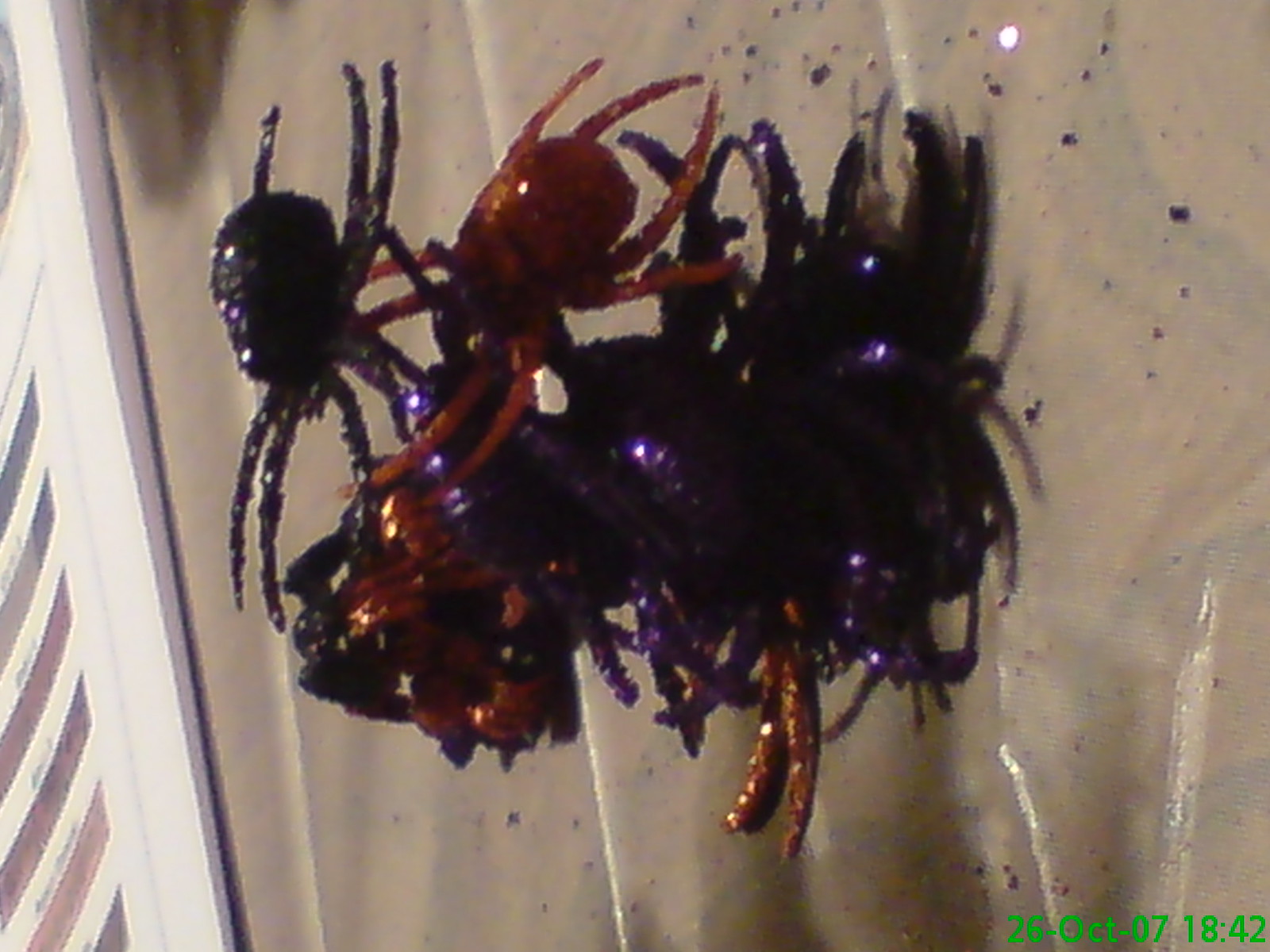The photograph, dated October 26, 2007, at 18:43, appears to be a collection of Halloween-themed plastic spiders, glistening with various colors and sprinkled with glitter. The spiders are a mix of black, purple, and dark orange, with some of them featuring purple sparkles. They seem to be somewhat floating above an uneven, possibly vinyl, beige surface, which could be a tablecloth or a piece of finger-painting paper covered with paint splotches. The scene is framed on the left by a white area with crossing lines and purple and white diagonal stripes. Lime green text in the bottom right corner of the image shows the timestamp. The entire setup gives the impression of festive Halloween decorations arranged in a dynamic, somewhat artificial manner, due to the unnatural positioning of the spiders’ legs and their shimmering appearance.